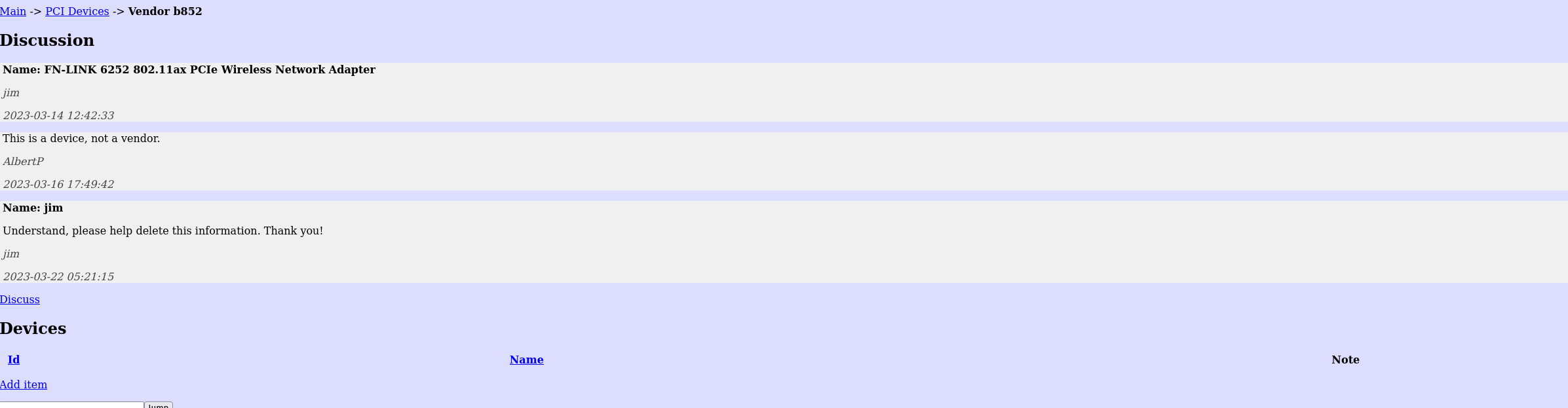This image is a small, rectangular graphic, significantly wider than it is tall. The background is primarily a regular shade of gray. The top left corner features the word "Discussion" in very small text. Below this, there are three columns stretching across with a very light gray background, containing various words that are difficult to make out due to their small size. In the bottom left corner, the word "Devices" is prominently displayed in black. Towards the center bottom, another small word is visible, as well as an additional word in the bottom right corner. The top left corner houses three very small words, with the first two in blue and the third in black. This intricate layout with varying text sizes and colors suggests a detailed document or interface layout, though the small text makes it challenging to discern specific details.